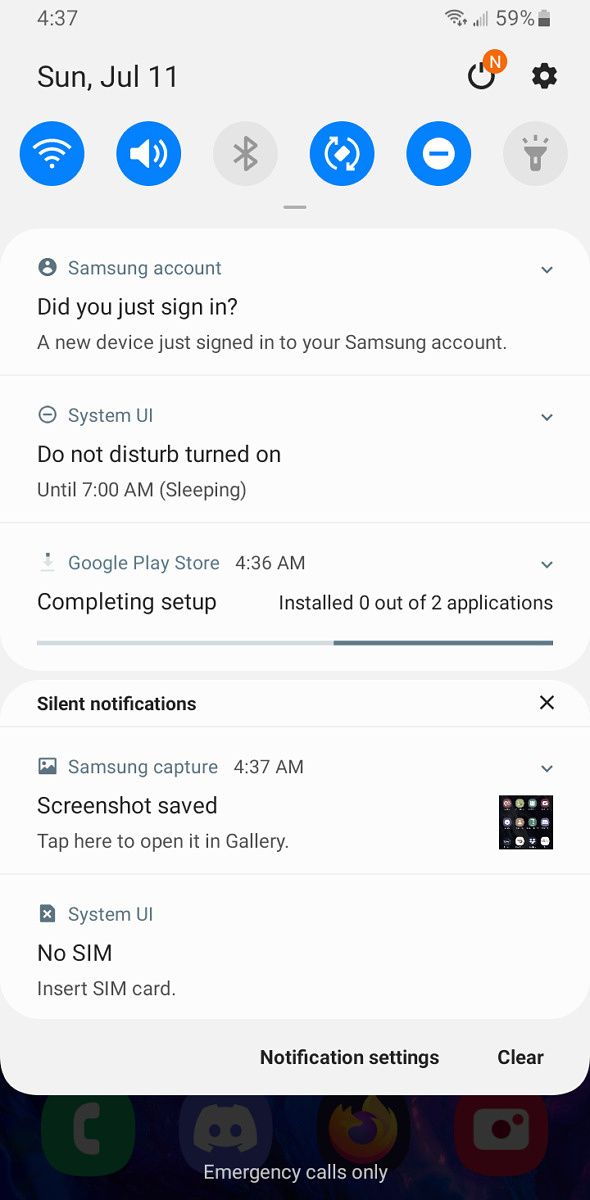Screenshot of a mobile phone taken on an Android device. At the top, there is a grey status bar displaying the following details: the time "4:37" in grey text, full WiFi signal, two bars of cellular service, and a battery icon showing 59% charge. The battery appears just over half full. Below, in black text on a white background, it says "Sunday, JUL 11". To the right, there is an icon for power settings depicted by an orange circle with a white "N" inside it, followed by a black gear icon representing options.

In the quick settings bar, blue icons indicate that WiFi, volume, and screen rotation are active. Bluetooth and the flashlight are inactive. Below this bar, on a white background with grey text, various notifications are listed:

1. "Samsung account: Did you just log in and do a nice or sunny day for your Samsung account."
2. "System UI: Do Not Disturb on until 7 AM, sleeping."
3. "Google Play Store: 4:36 PM, Completing update, 0 out of 2 applications."
4. "Silent Notifications: Samsung Capture, 4:37 AM, Screenshot saved. Tap here to open Gallery."
5. "System UI: No SIM, insert SIM card."

At the bottom of the screen, in black text, it says "Notification settings," and there are app icons for Phone, Discord, Firefox, and another unidentified app. At the bottom of the screen, it states "Emergency calls only" in white text.